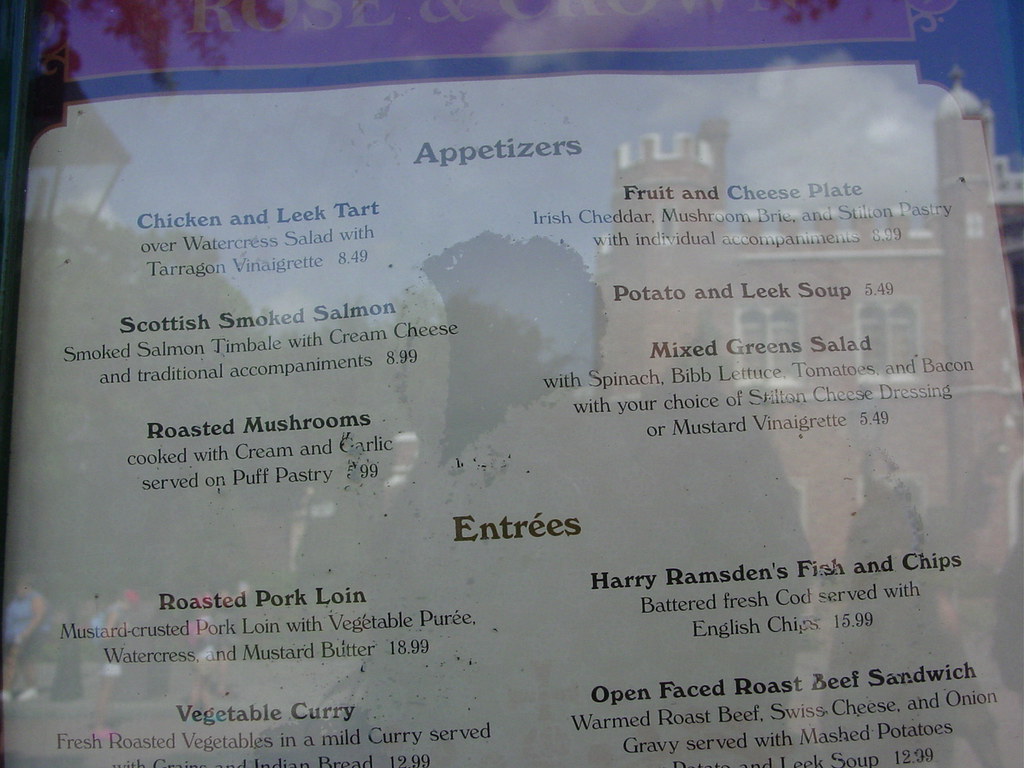This detailed photograph captures a menu displayed through a window, which reflects a building that resembles a church, identifiable by its architectural elements. Prominently seen is a red brick structure adorned with white molding and featuring a turret at the top. The second floor boasts distinctive arched windows, while the first floor appears to have squared-off windows.

The menu itself is titled "Rose and Crown" at the top, potentially hinting at the Rose and Crown restaurant located at Disney. For appetizers, the offerings include a Chicken and Leek Tart served over a Watercress Salad with Parmesan Vinaigrette priced at $8.49, a Fruit and Cheese Plate, Scottish Smoked Salmon for $8.99, Potato Leek Soup for $5.49, Mixed Green Salad for $5.49, and Roasted Mushrooms for $5.99.

The entrees listed are Roasted Pork Loin for $18.99, Harry Ramsden Fish and Chips for $15.99, Vegetable Curry for $12.99, and an Open-Face Roast Beef Sandwich for $12.99.